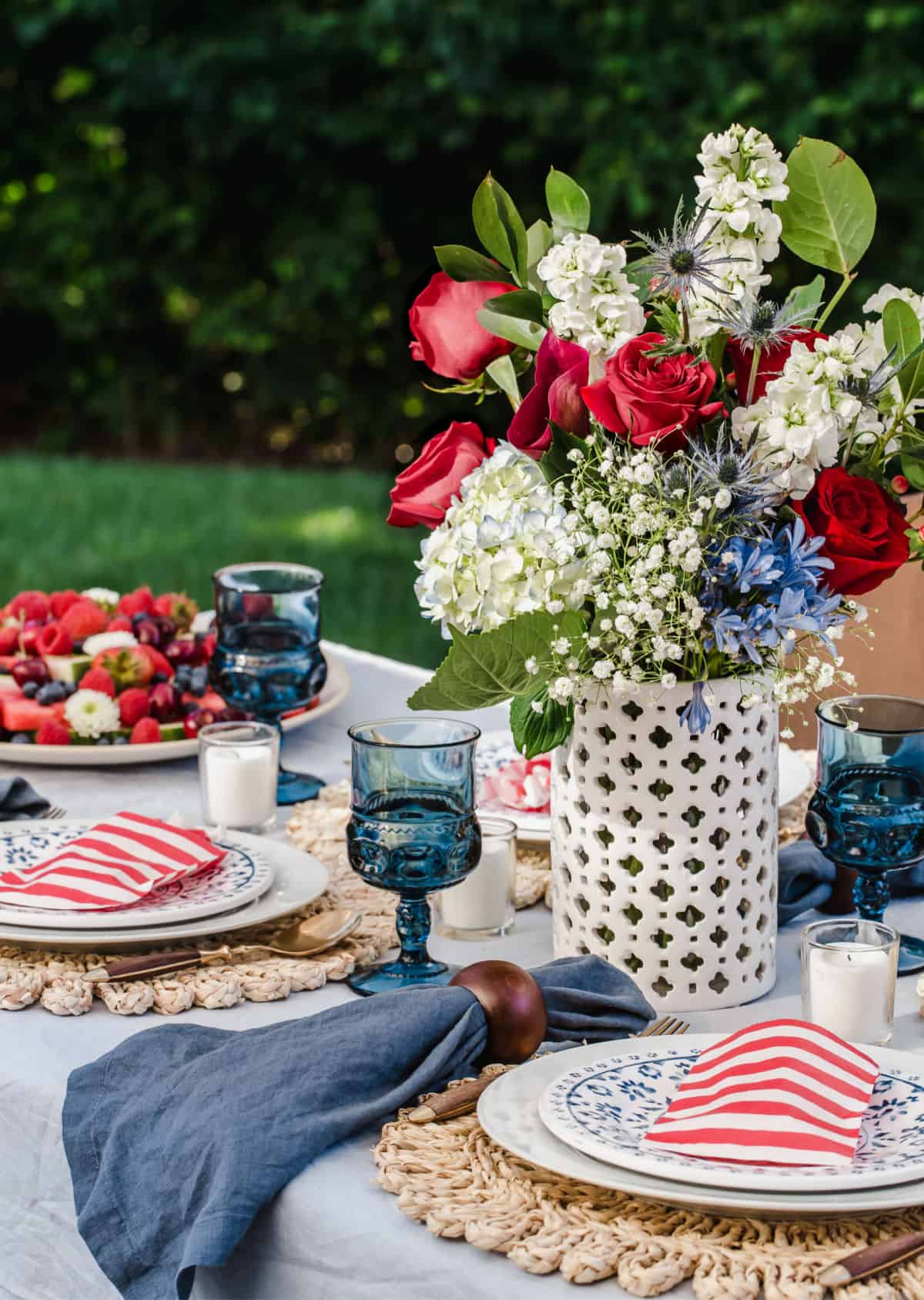The image captures an exquisitely decorated outdoor table setting, perfect for a festive 4th of July picnic. A white tablecloth drapes elegantly over the table, adorned with detailed crocheted placemats and matching table mats. The centerpiece is a vertical vase showcasing an impressive floral arrangement of red roses, white lilies, green leaves, and other ornamental touches. Flanking this are beautiful blueish-green goblets and pristine white candles in clear containers.

The table's dinnerware is equally striking, featuring a combination of blue and white plates— the smaller plates sitting atop larger ones, each decorated with blue floral patterns and topped with red-and-white striped napkins. Notable on the table is a blue napkin wrapped with a brown ring, adding a touch of rustic charm. In the background, there is a plate laden with fresh strawberries and blueberries, resembling a delectable strawberry shortcake dessert. The scene is perfectly framed by a soft-focus backdrop of manicured lawn, hedge line, and blurred trees, adding to the overall picturesque and patriotic ambiance.